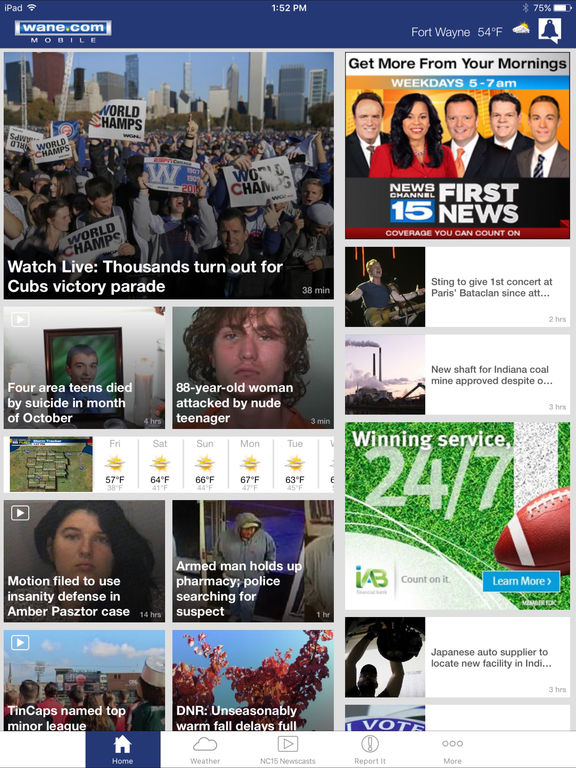Sure, here’s a cleaned-up and detailed caption for the image based on the voice description:

---

The vertical image is a screenshot taken from a smartphone device, capturing a page from a news website. At the top, the device interface indicates it is 1:52 PM, with symbols for Wi-Fi, Bluetooth, and a battery life of 75%. The header also shows the device name, 'Wayne Comm and Memorial Mobile,' and the local weather report for Fort Wayne, which is currently 54 degrees with a sun-cloud icon. Adjacent to these details is a notification bell icon.

Below the header is a promotional banner stating, "Get more from your mornings, weeks, days 5 to 7 a.m.," featuring photos of the newscasters from News Channel 15 and the slogan, "First news coverage you can count on." To the left of the news team images, a prompt mentions the option to watch live coverage of thousands turning out for the Cubs victory parade.

Further down the screen, there are several clickable articles, a map, and an extended weather forecast for the next several days. Additional articles are listed below the newscasters' photos with headings that denote more content available for readers. At the bottom, a service slogan reads, "Winning service 24/7 you can count on it. Learn more."

Finally, the navigation bar at the bottom of the screen highlights the 'Home' tab in blue, with other clickable options including 'Weather,' '15 Newscasts,' and more.

---

This refined caption provides a comprehensive and organized description of the image.